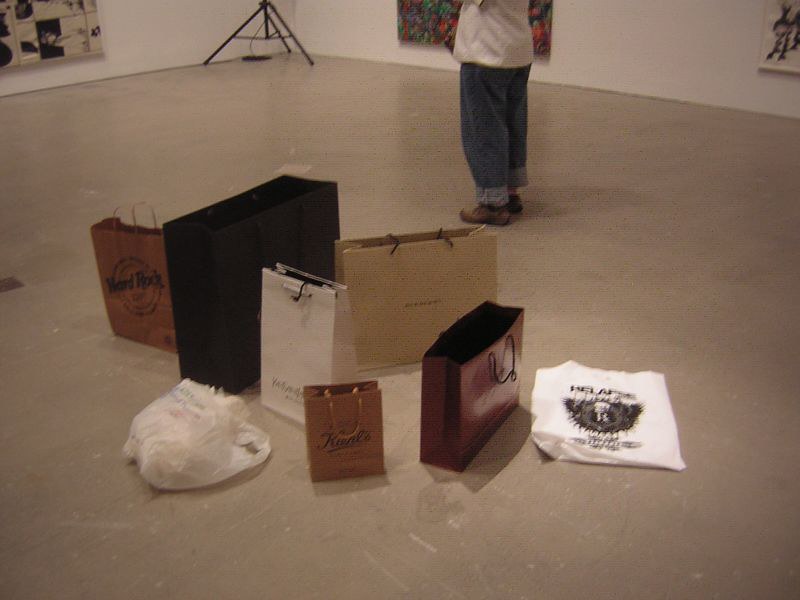The image captures the floor of what appears to be an art gallery, displaying a polished grey surface with white marks that reflect the lighting subtly. Scattered prominently in the center of the floor are several high-quality shopping bags of various sizes and colors, including brown, black, white, beige, and red. These bags, featuring logos such as Hard Rock Cafe and Kiehl's, sport the telltale rope handles often associated with upscale retail purchases. Along the back right and extending to the left at a 90-degree angle are white walls adorned with large canvas paintings. One artwork, visible slightly off-center, is a vibrant, multicolored piece, while another on the left features a stark black-and-white design. Slightly to the right and higher in the frame, the legs and torsos of a person dressed in blue jeans, brown shoes, and a white top or jacket can be seen, adding a human element to the otherwise still scene. The overall atmosphere of the image suggests a low-light, slightly grainy quality, reinforcing the serene and introspective environment of the gallery.